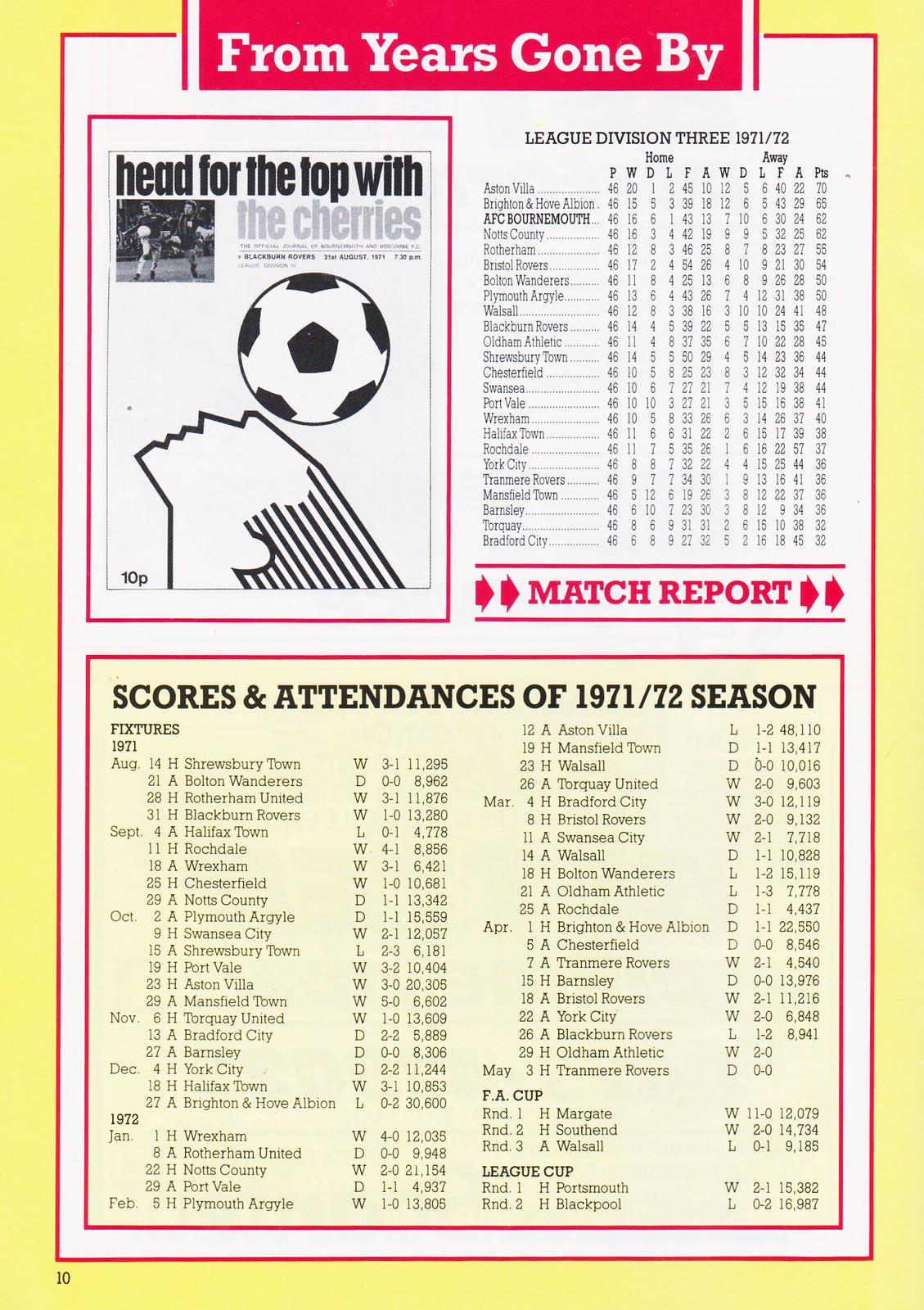The tall rectangular image depicts a page from a sports program with a bright yellow pastel border. At the top, a bright red rectangle, overlapping the pastel border, reads "From Years Gone By" in white font. Below this, the page is divided into three sections on a white background. 

On the left side, there is an advertisement for another program titled "Head for the Top with the Cherries," priced at 10p. This advertisement features an illustration of a person heading a soccer ball. Adjacent to this, the right section displays the header "League Division 3, 1971-72" in red, along with lists of various teams with their respective home and away statistics.

At the bottom of the page, in a pale yellow rectangle traced by a red line, a table summarizes the "Scores and Attendances of 1971-72 Season" in bold, capitalized, black letters. This section appears to provide a comprehensive schedule spanning from August 1971 to May 1972, detailing wins, losses, draws, and attendance records for different teams. Additionally, the page number "10" is indicated at the bottom, suggesting this is page ten of the program.